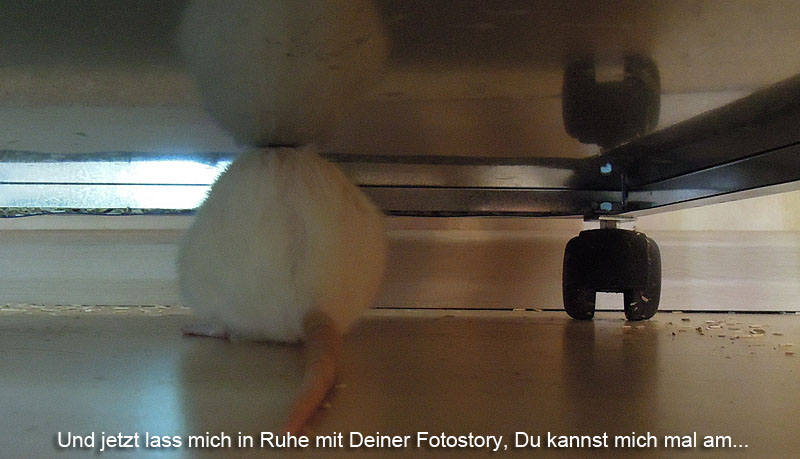The photograph captures a scene from a low, ground-level perspective, as if the camera is positioned directly on the floor. It appears to be taken from underneath a piece of furniture resembling a bed with black wheels and metal supports, possibly made of aluminum, as well as a reflective metal bottom. The floor beneath is a wood-like brownish-yellow, scattered with debris resembling shredded wood chips or animal bedding.

In the center, the focus is on the back side of a white rat, showcasing its pink tail and part of its left foot. The rat seems cornered with its face pressed against the white-painted wall and baseboard trim, creating an impression of it seeking refuge. The setting is further defined by the presence of a slightly reflective metal underside of the furniture, which faintly mirrors the rat's silhouette.

Along the bottom edge of the photograph, white text spans from the left corner to the right, written in a foreign language that adds an intriguing, international element to the scene. The ambient light subtly filters in, casting a gentle illumination that emphasizes the hidden, almost secretive nature of the view under the furniture.